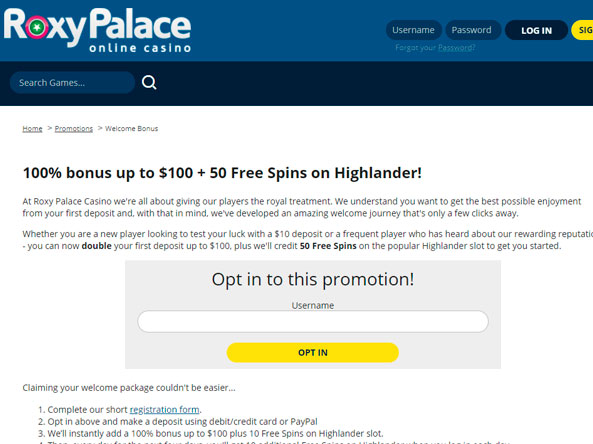**Roxy Palace Online Casino Welcome Screen**

The image depicts a screenshot of the Roxy Palace Online Casino's welcome screen. In the upper left-hand corner, the casino's logo is prominently displayed. On the upper right-hand portion, there are fields for entering a username and password, accompanied by a login button. Additionally, a partially visible sign-up button is situated next to the login button.

Beneath this section, on the left side of the screen, is a search bar labeled "Search games." Below the search bar, several navigational links are listed: "Home," "Promotions," and "Welcome Bonus."

A significant highlight is the promotional offer detailed on the screen. Players are greeted with a welcome bonus of 100% match on their first deposit up to $100, along with 50 free spins on the Highlander slot game. The promotional text emphasizes Roxy Palace Casino's commitment to providing players with a royal treatment and an enjoyable gaming experience. New players are particularly encouraged to take advantage of this offer, whether they are making a $10 deposit or looking to maximize the bonus.

Further down, the screen features a section prompting players to opt into the promotion. There is a text box for entering a username, followed by a conspicuous yellow "Opt-In" button with black text, inviting players to participate in the promotional offer.

The overall presentation is inviting and clearly designed to encourage new and existing players to engage with the casino's offerings and incentives.